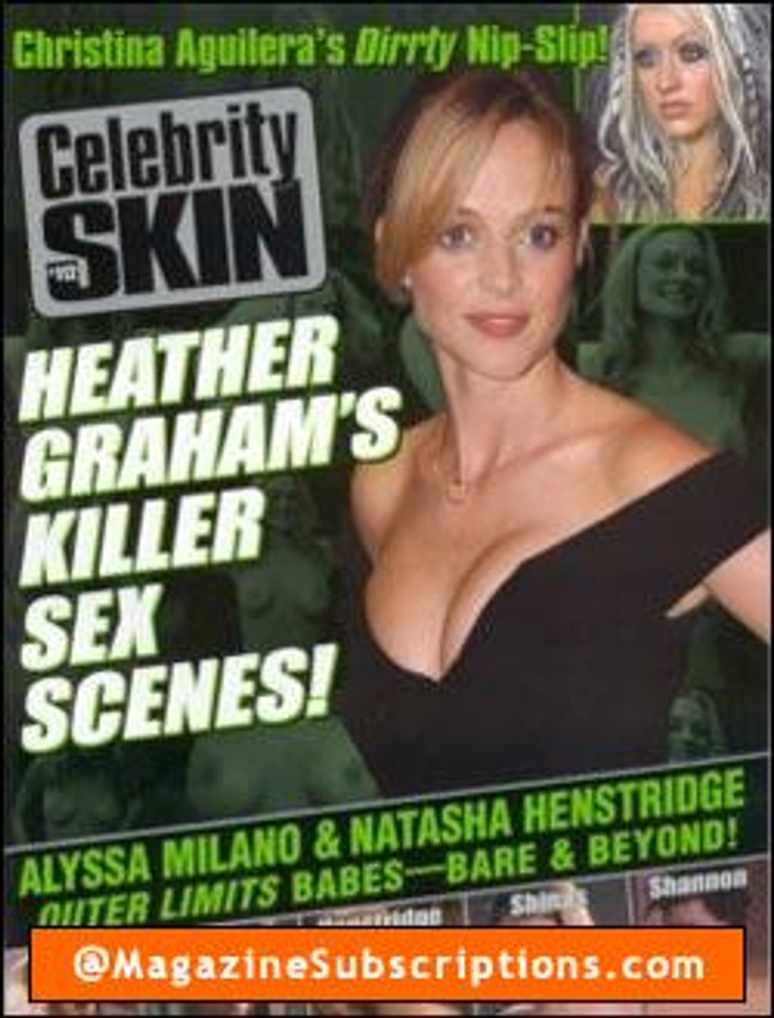This image features a slightly low-definition magazine cover for "Celebrity Skin," likely from the early 2000s. The title "Celebrity Skin" is prominently displayed in a black font on a gray box in the upper left corner. Dominating the right side of the cover is a young blond woman with hair pulled back, wearing a low-cut black dress with one strap hanging off her left shoulder. She is slightly smiling but not looking directly at the camera. In the upper-right corner, there is a close-up photograph of Christina Aguilera with her name headlined across the top, "Christina Aguilera's Dirty Nip Slip."

Towards the center of the cover, bold white capital letters announce "Heather Graham's Killer Sex Scenes." Below this, a diagonal banner reads, "Alyssa Milano and Natasha Henstridge, Outer Limits Babes, Bare and Beyond." The background features grainy, green-and-black images resembling night-vision footage, showing partially exposed women. An orange banner at the bottom of the cover advertises "At Magazine Subscriptions Dot Com."